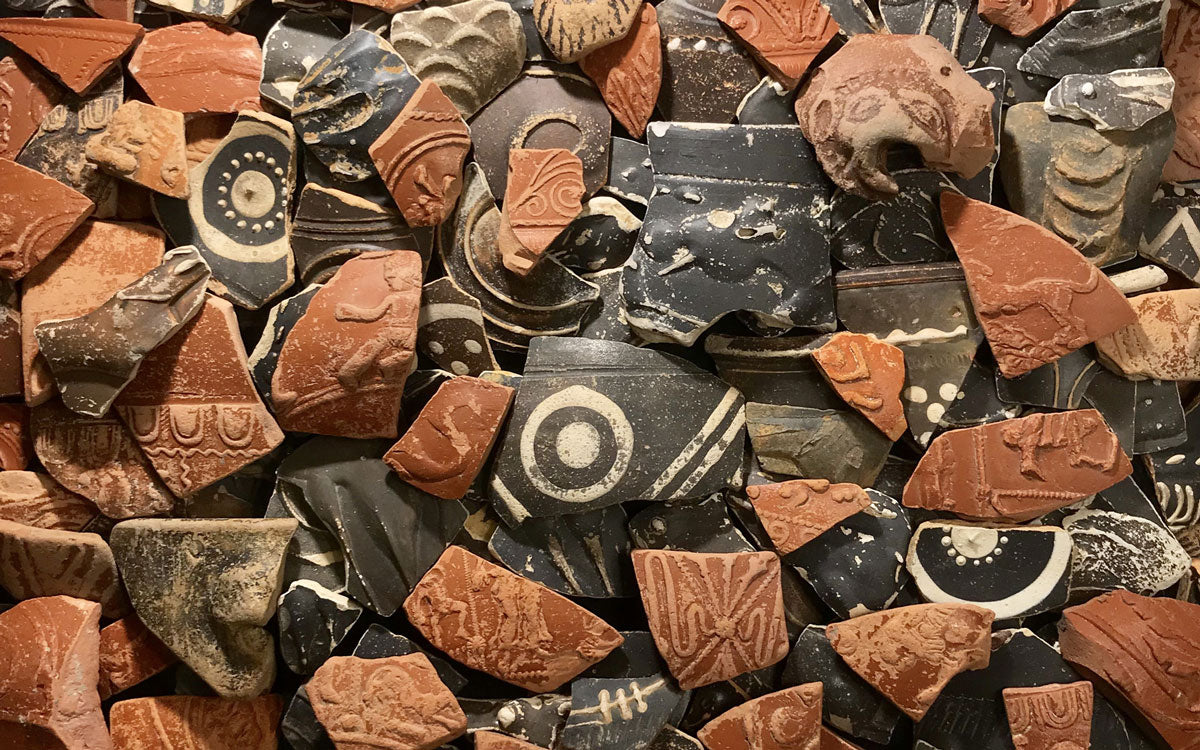Captured in a full-color photograph under artificial lighting, this horizontally rectangular image showcases an assortment of broken pottery shards. The collection, likely several dozen pieces, includes terracotta-colored fragments adorned with intricate designs. These designs depict animals, people, and architectural patterns, possibly evoking the hieroglyphic art of ancient civilizations. Some pieces are gray or stone-like, appearing rougher and older compared to the others, yet still bearing carved designs. A striking feature among the pottery is the jet-black shards decorated with white paint in circular and sun-like patterns. The shards are piled together, some overlapping, creating a complex mosaic of ancient artifacts that hint at a rich historical past.